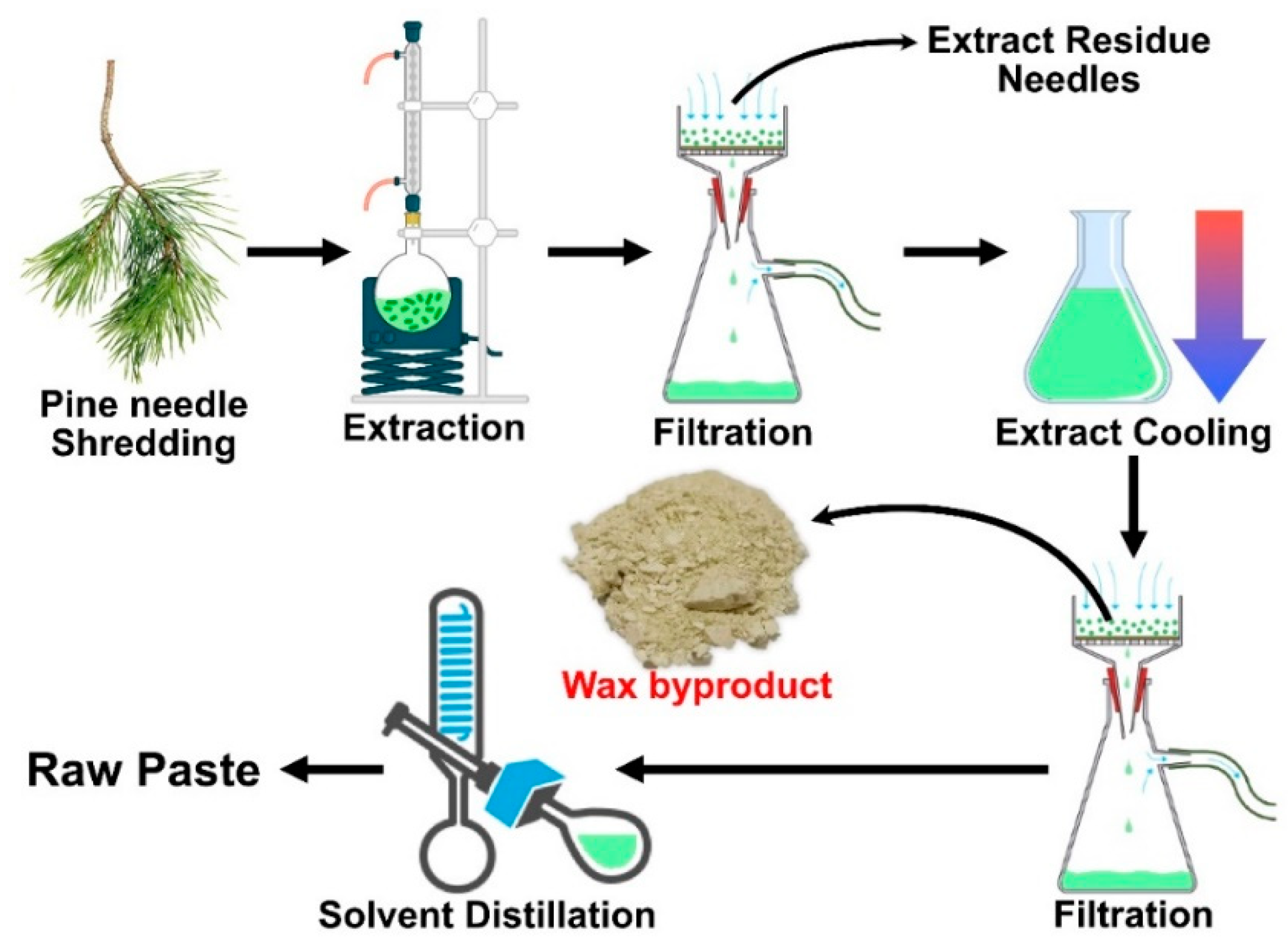The diagram illustrates a detailed experimental process in chemistry, depicted in a sequential flow. Starting at the top left, a photograph shows a pine branch with needles labeled "pine needle shredding." Moving right, a black arrow leads to an image of a round-bottom flask containing green liquid and particles, labeled "extraction." This flask is mounted on a tall, silver apparatus. Next, a beaker features blue arrows indicating a downward flow of the same green substance, alongside red elements dripping green liquid, labeled "filtration."

A black arrow pointing upward labels the residue as "extract residue needles," which then leads to another flask containing green liquid. A red-to-purple-to-blue gradient arrow points downward towards the text "extract cooling." Below this, multiple blue arrows direct the flow back to green dots in a repeated manner, labeled "fermentation," followed by another black arrow and text "wax by-product" beneath it in red, indicating a brown powder.

The final stage features a large black arrow pointing towards "solvent distillation," culminating in the creation of "raw paste." Throughout the image, various chemistry apparatuses such as beakers and flasks are depicted, and key steps are marked with textual labels and color-coded arrows, illustrating the entire transformation from pine needles to raw paste with intermediary steps like extraction, cooling, and by-product formation.